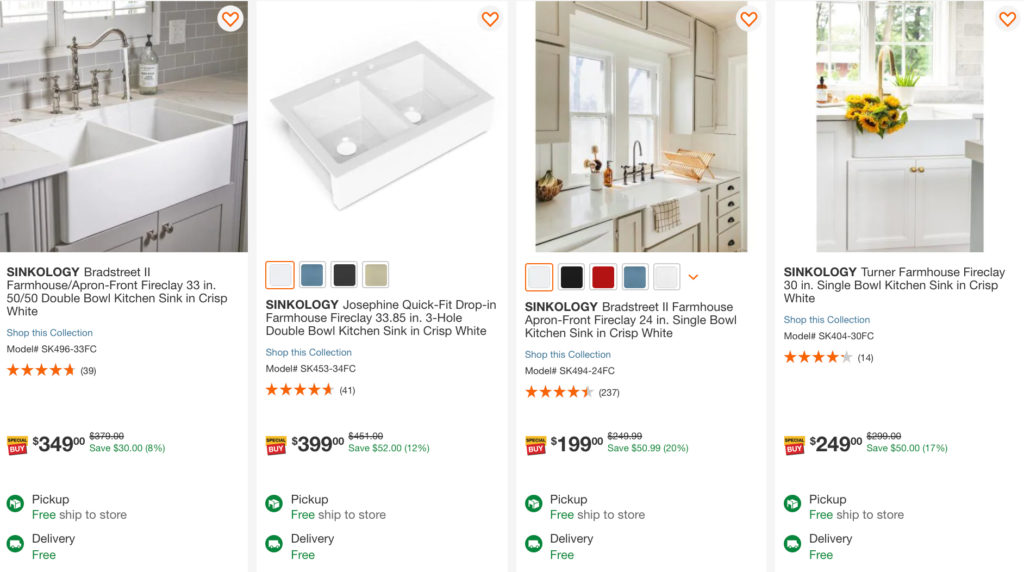This image showcases the product sections of an online shop, specifically focusing on various farmhouse kitchen sinks. Here's a detailed description of the four featured sinks:

1. **Sinkology Bread Street 2 Farmhouse Apron-Front Fireclay 33-Inch Double Bowl Kitchen Sink in Crisp White**:
   - **Features**: Mounted between cabinets, this 33-inch double bowl sink boasts an elegant, crisp white finish. 
   - **Ratings**: 5-star rated by 39 customers, with ratings displayed in orange.
   - **Pricing**: Priced at $349, marked down from the original $379, offering savings of $30 (approximately 8%).
   - **Additional Details**: Highlighted as free pickup, free ship-to-store, and free delivery options available. 

2. **Sinkology Just Fine Quick-Fit Drop-In Farmhouse Fireclay 33.85-Inch Three Hole Double Bowl Kitchen Sink in Crisp White**:
   - **Features**: This sink, which fits easily into farmhouse-style kitchens, comes in a larger 33.85-inch size with three holes.
   - **Ratings**: Receiving high praise, it holds a 4.9-star rating.
   - **Pricing**: Currently priced at $399, reduced from $451, saving customers $52 (around 12% savings).
   - **Color Options**: Selectable in grey, dark blue, black, and brown.

3. **Sinkology Bread Street 2 Farmhouse Apron-Front Fireclay 24-Inch Single Bowl Kitchen Sink in Crisp White**:
   - **Features**: A smaller 24-inch single bowl variant, this sink features the same stylish crisp white look.
   - **Ratings**: Holds a 4.5-star rating.
   - **Pricing**: Discounted to $199 from $249.99, offering savings of $50.99 (approximately 20%).

4. **Sinkology Turner Farmhouse Fireclay 30-Inch Single Bowl Kitchen Sink in Crisp White**:
   - **Features**: A mid-size option at 30 inches, this sink provides a spacious single bowl in crisp white.
   - **Ratings**: Rated 4.1 stars.
   - **Pricing**: Offered at $249, down from $279.99, saving $30 (about a 17% discount).

The sinks are all high-quality fireclay models, promoting durability and style, with multiple pricing options and significant savings.